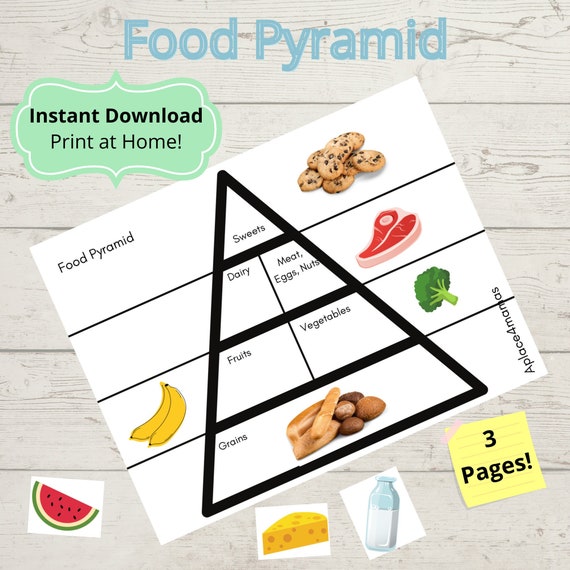This illustration appears to be an informational poster of a food pyramid like you might find on a web page or in a health book. The title "Food Pyramid" is written in light blue font at the top. Below the title, there's a small bubble that says "Instant Download, Print at Home." The food pyramid is depicted on a white board with a black outline. 

The pyramid is divided into several levels: 
- At the top level labeled "Sweets," there's a picture of chocolate chip cookies.
- The next level down is labeled "Dairy," and beside it are "Meat, Eggs, Nuts," accompanied by an image of a steak.
- Moving further down, the "Fruits and Vegetables" level features illustrations of a banana on the left and broccoli on the right.
- At the base of the pyramid, labeled "Grains," there are various types of bread and rolls.

In the background at the bottom of the image, surrounding the pyramid, there are additional pictures of a watermelon, a piece of cheese, and a milk bottle. A yellow sticky note nearby states "Three Pages!" The overall look gives a neat, organized feel with informative and easy-to-understand visuals, making it suitable for educational purposes or web content.